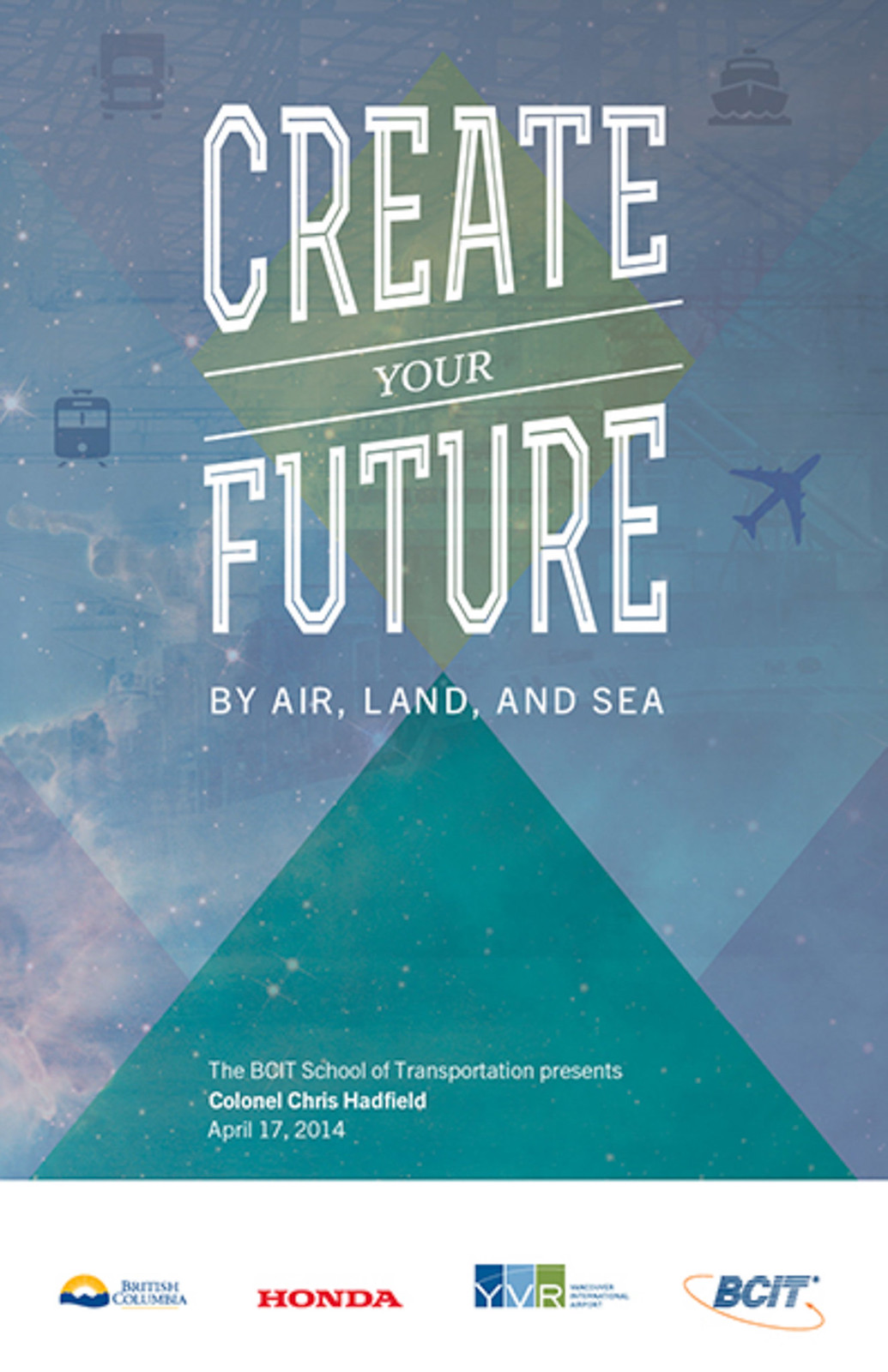The poster features a blue rectangular background with varying hues of blue, accentuated by a starry backdrop. Dominating the top portion is a light green diamond shape, and at the bottom, there is a brighter green upward-pointing triangle. Prominently displayed in large white text at the top is the phrase "Create Your Future by Air, Land, and Sea." In the top and middle sections of the poster, icons of various modes of transportation are showcased: a bus, a tram, a ferry, an airplane, a truck, a boat, and a train, indicating diverse transport mediums.

Below the transport icons, the text "The BCIT School of Transportation presents Colonel Chris Hadfield, April 17, 2014" is displayed. The bottom of the poster features logos of the event sponsors, including Honda, YVR, British Columbia, and BCIT. The detailed layout and text suggest it is likely a promotional poster for a transportation-themed event or presentation.